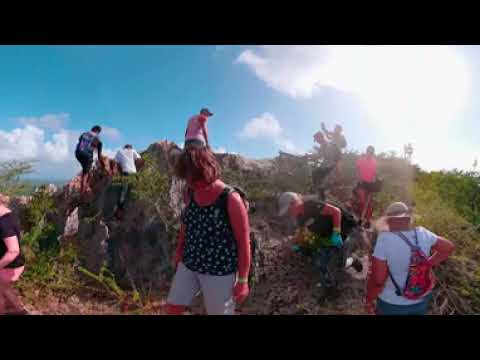The image shows a group of predominantly white-skinned tourists, mostly women with a few men, hiking on a grassy hillside under a warm, sunny blue sky with scattered clouds. Everyone is dressed in short summer clothing, with many wearing hats or baseball caps and some donning rubber gloves and backpacks. The terrain includes dirt, grass, and weeds, and features a noticeable rock outcropping toward which several people are climbing or walking. Notably, one woman at the center of the image appears to be getting sunburned. The sunny day and the group’s attire suggest a warm climate, and the presence of long horizontal black bars at the top and bottom indicate the image might be a screen capture from a video.